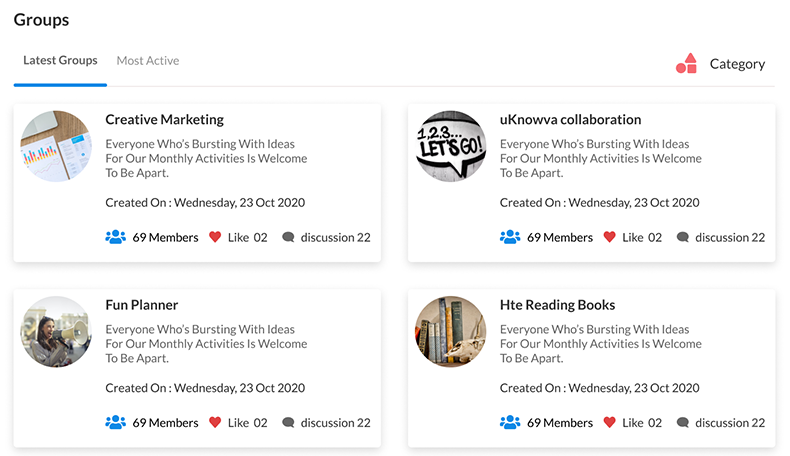The webpage features a clean, white background. In the top left corner, the word "Groups" is prominently displayed in bold black lettering. Below it, slightly smaller and still in bold black, is the label "Latest Groups". To the right of "Latest Groups" in gray typography is "Most Active". On the right side of the page, there is a vertical sequence of shapes: a red circle, a red square, and above the square, a red triangle. Adjacent to these shapes is the word "Category" in black text.

Under the "Latest Groups" section, a blue line extends across the page, transitioning into a thin gray line near the "Most Active" label.

Four equally-sized white rectangular tabs are arranged in a grid, with a thin gray border encircling each tab. Each tab has a profile picture circle in the top left corner, followed by the name of the group in bold black text. The groups are as follows:
1. Top Left: "Creative Marketing"
2. Bottom Left: "Fun Planner"
3. Top Right: "Group Title 3" (implied but not described in the provided text)
4. Bottom Right: "Group Title 4" (implied but not described in the provided text)

Beneath each group name, two and a half lines of descriptive information are provided. Further down, the creation date "Wednesday 23rd October 2020" is noted.

Icons and statistics for each group are consistent, featuring:
- A blue icon with three profile silhouettes followed by "67 members" in black text.
- A red heart icon with "02" in black text.
- A black discussion icon with "Discussion 22" in black text.